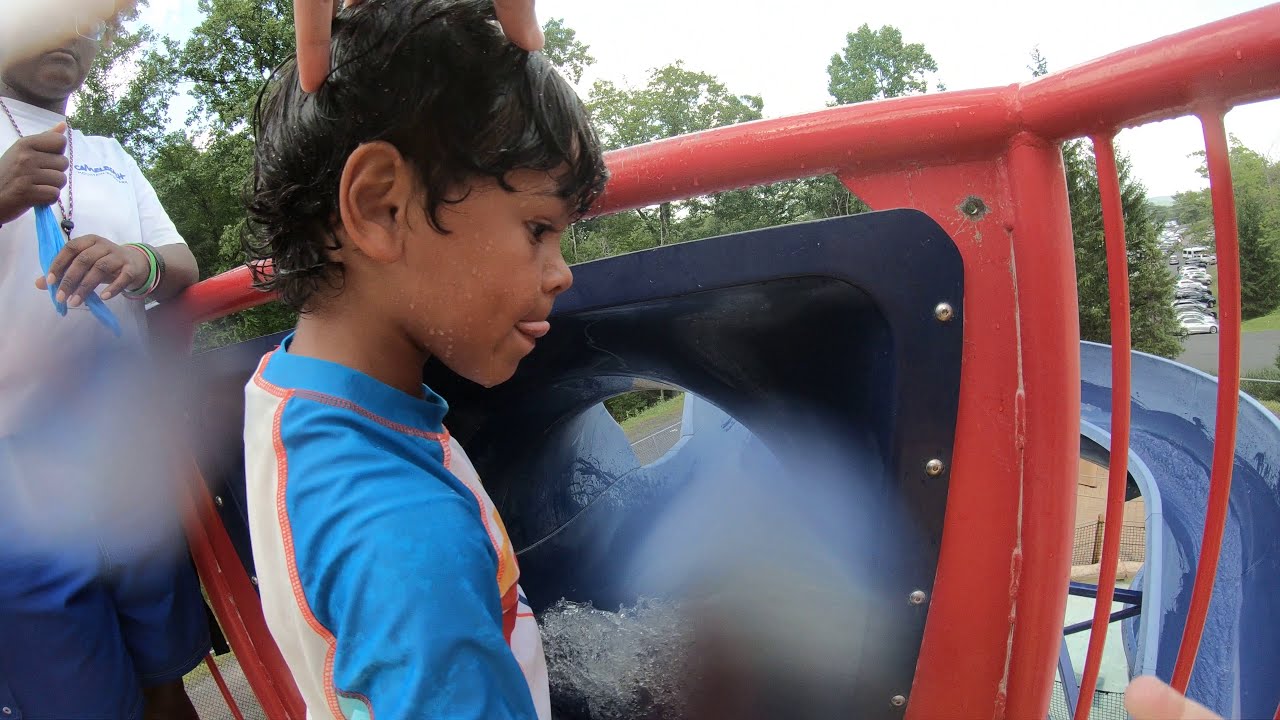The image captures a lively scene at a playground featuring a young boy who appears to be around six years old. He stands at the entrance of a small blue water slide, which is wet and glistening with splashes. The boy, with curly black hair, wears a blue and white swim shirt and has water droplets on his face. He's playfully licking his upper lip while standing in front of the slide. The background shows an adult in a white shirt, possibly a supervisor, carrying a whistle or lanyard. There are blurred spots in the image, likely due to water on the camera lens. Trees and the metal and plastic structures of the playground complex can be seen in the background, adding to the vibrant outdoor setting.